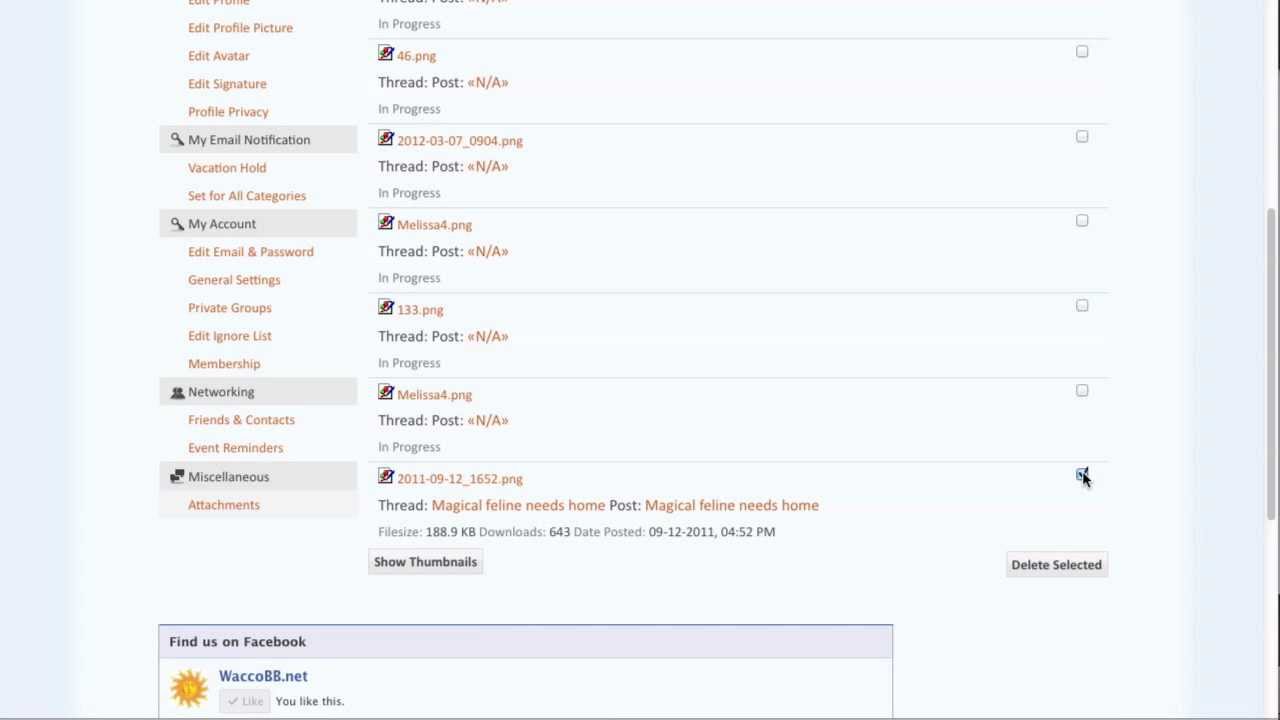A partial screenshot of a website page predominantly featuring a user profile and settings menu. The top of the page is cut off, resulting in some text being partially obscured. On the left side of the screen, there is a navigational menu with several options displayed in orange and black text. The options include "Edit Profile Picture," "Edit Avatar," "Edit Signature," and "Edit Privacy" in orange. Following these, in black, are "My Email Notifications" and, in orange again, "Vacation Hold Set for All Categories." 

Continuing down, the section labeled "My Account" appears in black, with sub-options like "Edit Email and Password," "General Settings," "Private Groups," "Edit Ignore List," and "Membership." The next section, labeled "Networking," includes "Friends and Contacts" and "Event Reminders," highlighted in orange. The last section, "Miscellaneous," features the option "Attachment" highlighted in red or orange.

In the main content area of the page, several entries are listed, identifying different PNG files that appear to be related to forum threads or posts. These include:
- "46.PNG Thread Post NA In Progress, 2012-03-07-09-04"
- "Ping Thread Post NA In Progress, Melissa4.PNG Thread Post NA In Progress, 2013.PNG Thread Post NA In Progress, Melissa4.PNG Thread Post NA In Progress, 2011-09-12-16-52"
- "Ping Thread Magical Feline Needs Home, Post Magical Feline Needs Home."

One particular entry details a file called "Magical Feline Needs Home," showing attributes such as file size (188.9 KB), number of downloads (643), and the date posted (09-12-2011 at 4:52 PM). There is also an option to "Show Thumbnails."